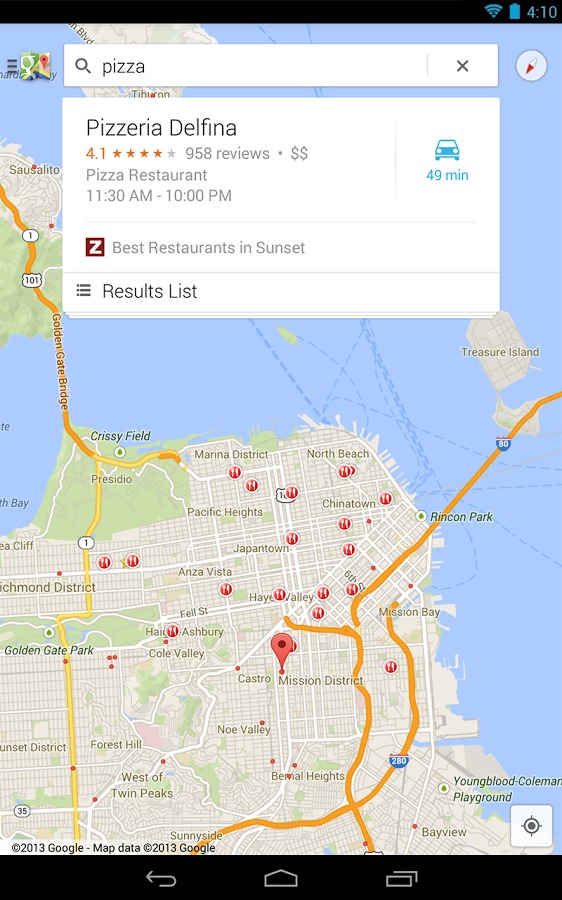This image is a detailed screenshot of a map application displayed on a smartphone. The interface includes thin black bars at the top and bottom of the screen. In the top right corner of the upper black bar, there are icons indicating a strong Wi-Fi signal, a fully charged battery, and the current time displayed as 4:10. The bottom black bar contains navigational icons for back, home, and tasks, represented by a left arrow, a circle, and a square, respectively.

Dominating the screen is a densely labeled map, primarily featuring a central landmass with extensive surrounding water areas. Two bridges extend from the top left and top right of this landmass. Prominent locations marked on the map include Japantown, Pacific Heights, Marina District, Crissy Field, Rincon Park, West of Twin Peaks, Youngblood Coleman Playground, Mission District, Chinatown, North Beach, and Treasure Island. 

At the top center of the image is a white search bar reading "pizza." Below this search bar, there is a white rectangular information box displaying details about a specific restaurant named "Pizza Delfina." It indicates a rating of 4.1 out of 5 stars based on 958 reviews and signifies the price range with two dollar signs ($$). The restaurant's operating hours are listed as 11:30 a.m. to 10 p.m., along with a note that it is among "The Best Restaurants in Sunset." A blue car icon is also visible, suggesting the travel time to the location is 49 minutes.